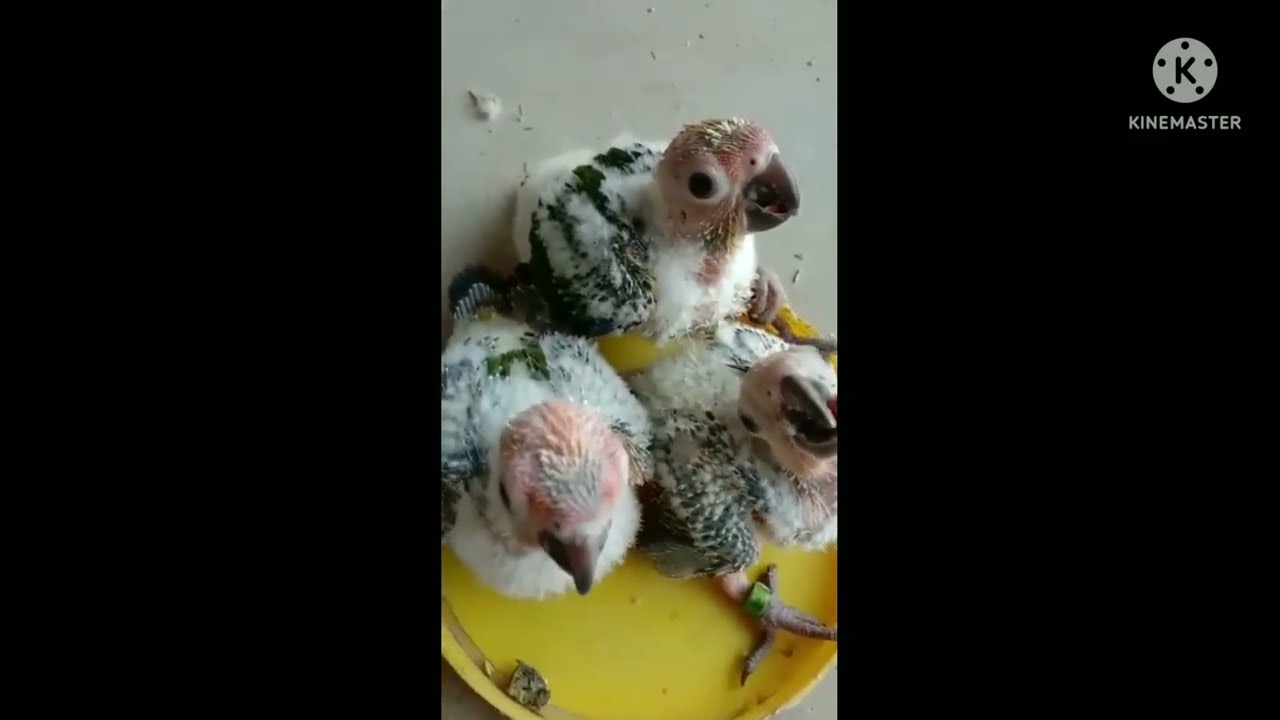The image portrays an overhead shot of three recently hatched chicks that resemble buzzards or vultures. They huddle together on a yellow platform, possibly a bucket, with their distinct pink heads, large white eyes with black centers, and black beaks standing out. Their bodies are primarily white with sparse black feathers. The scene is set against a white floor with a bright natural light source illuminating from the right. The central photograph has an aspect ratio higher than it is wide, resembling a cell phone's shape, and is framed by thick black borders, making the overall image wider than it is tall. In the upper right corner of the black border, the "KineMaster" logo is visible, featuring gray letters with a circular emblem containing a 'K' and some black dots.